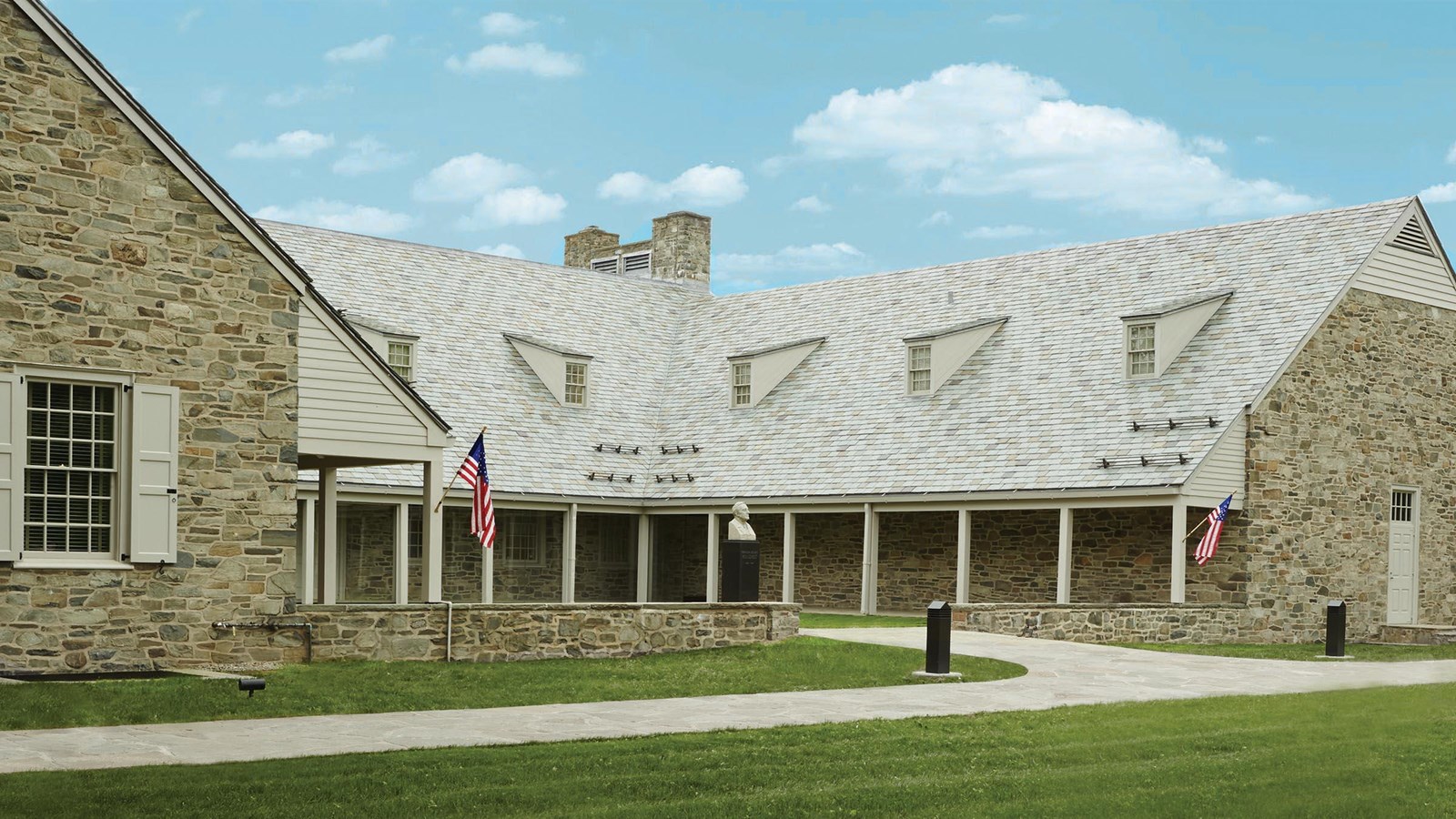This image depicts a stately, American-style building characterized by its classic architectural features and historical significance. The building, constructed with ashy brown-grey bricks, showcases white shutters and a beige roof adorned with a series of dormers, giving it a ranch-residential appeal despite its commercial or public nature. The structure forms a U-shape with two prominent gabled ends connected by an L-shaped section, against a backdrop of vibrant blue sky dotted with a few clouds. Two American flags flank the building, attached to the wooden frame that extends from the roof to the floor, symbolizing its patriotic essence.

In the courtyard, a marble bust of an unidentified historical figure rests on a black pedestal, reinforcing the building's link to important historical or cultural heritage. The scene is framed by a pristinely manicured lawn and neatly maintained surroundings, indicative of the building's well-preserved and protected state. Several informational podiums are present, though their content remains unreadable. The overall setting, devoid of people and bathed in pleasant weather, exudes a tranquil and venerable atmosphere.